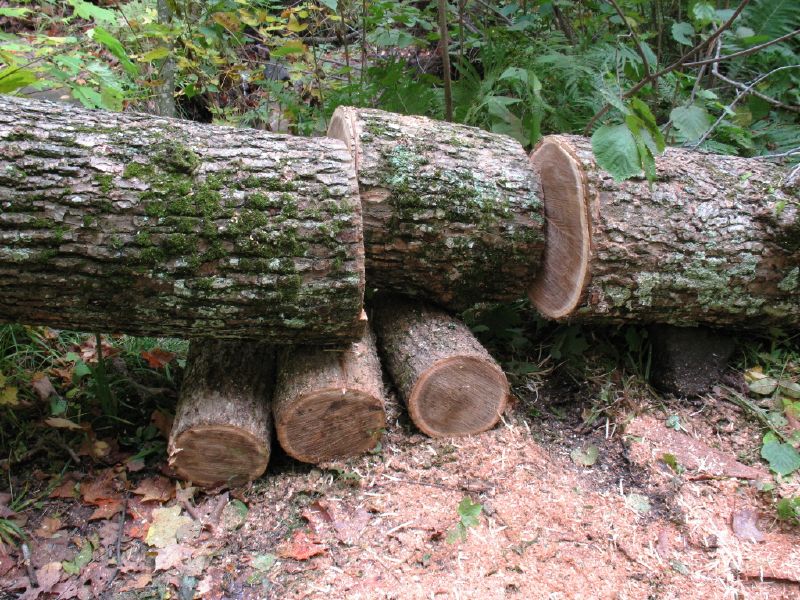In this detailed outdoor image of a woodland area, we see the scene set against a backdrop of varying shades of green foliage, interspersed with lighter greens, medium greens, and darker greens, along with an assortment of twigs and tree limbs. Yellow and brown leaves add splashes of autumnal color. Dominating the foreground is a sizable tree trunk, roughly cut into three uneven sections with the middle piece being the shortest. The horizontally positioned trunk segments reveal the texture of the wood's interior, with sawdust scattered beneath. Smaller logs, suitable for firewood, lay beneath the larger trunk, amidst fallen leaves and wood shavings. The ground underneath is a mix of dirt and sparse patches of short grass, highlighting the natural, untamed aspect of this scene which lacks indications of being a maintained yard, reinforcing its wild, forest-like quality.